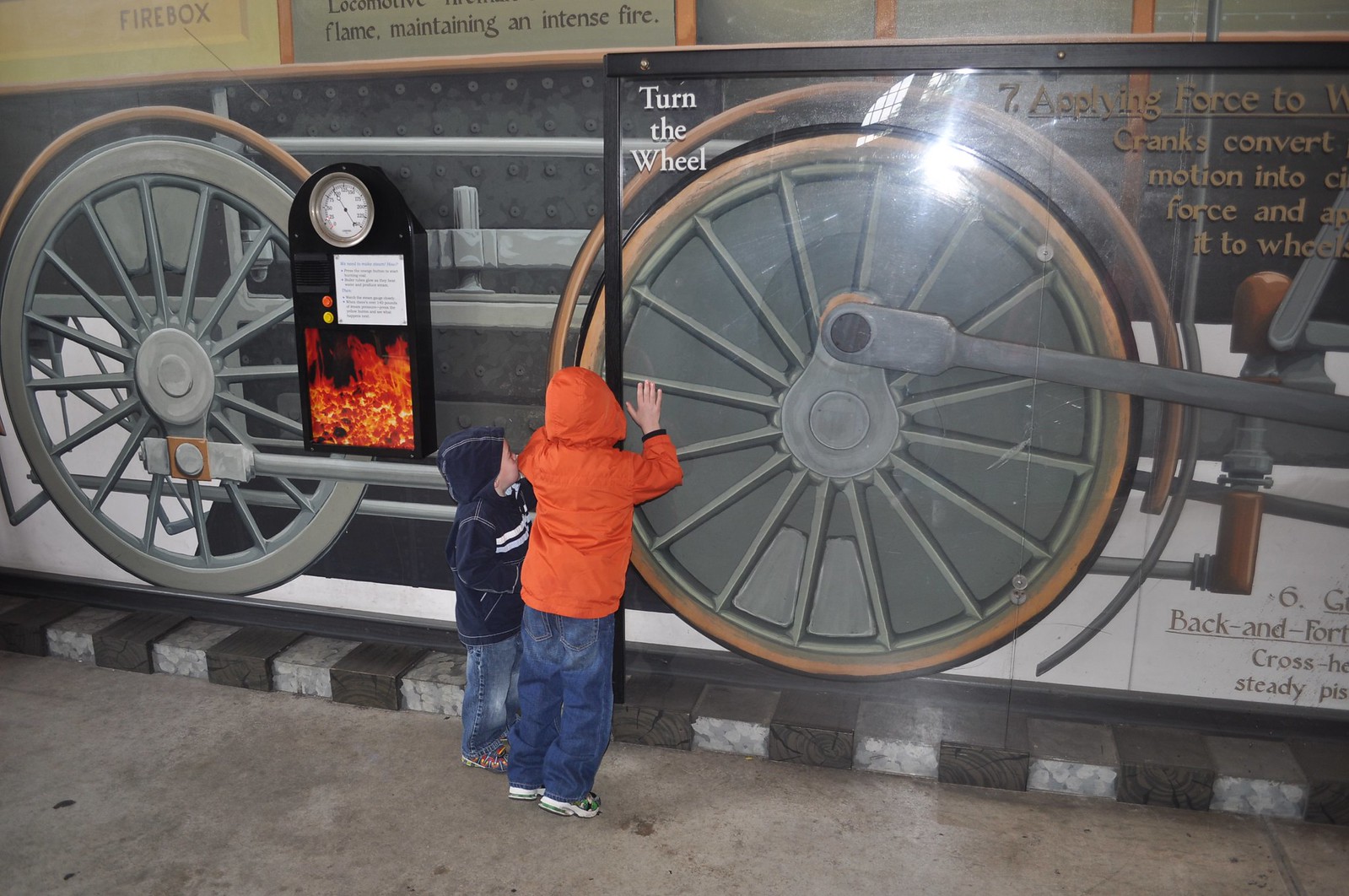The photograph captures two young boys engaged with a hands-on exhibit at what appears to be a museum, possibly a children's or science museum with a train theme. The boys, one wearing an orange jacket and the other a dark blue sweatshirt with white stripes, both clad in jeans, have their backs to the camera as they interact with a display featuring two illustrated train wheels. The child in the orange jacket, estimated to be around six or seven years old, is actively turning one of the wheels, which has spokes and is gray in color, guided by the text above it that reads "Turn the wheel." 

To the right of the boys, additional exhibit text is partially visible, stating, "applying force to" and "cranks convert motion into force," along with fragments such as "back and forth" and "steady." This text suggests an educational focus on mechanical principles. Adjacent to the interactive wheels is another part of the exhibit displaying a steam gauge and a panel with red flame imagery. The wheels are seemingly attached to a cart positioned on a brick platform, and the boys are standing on a cement surface. The upper part of the image features a gray poster with text including "flame," "maintenance," and "intense fire," reinforcing the display's thematic elements related to trains and mechanics.